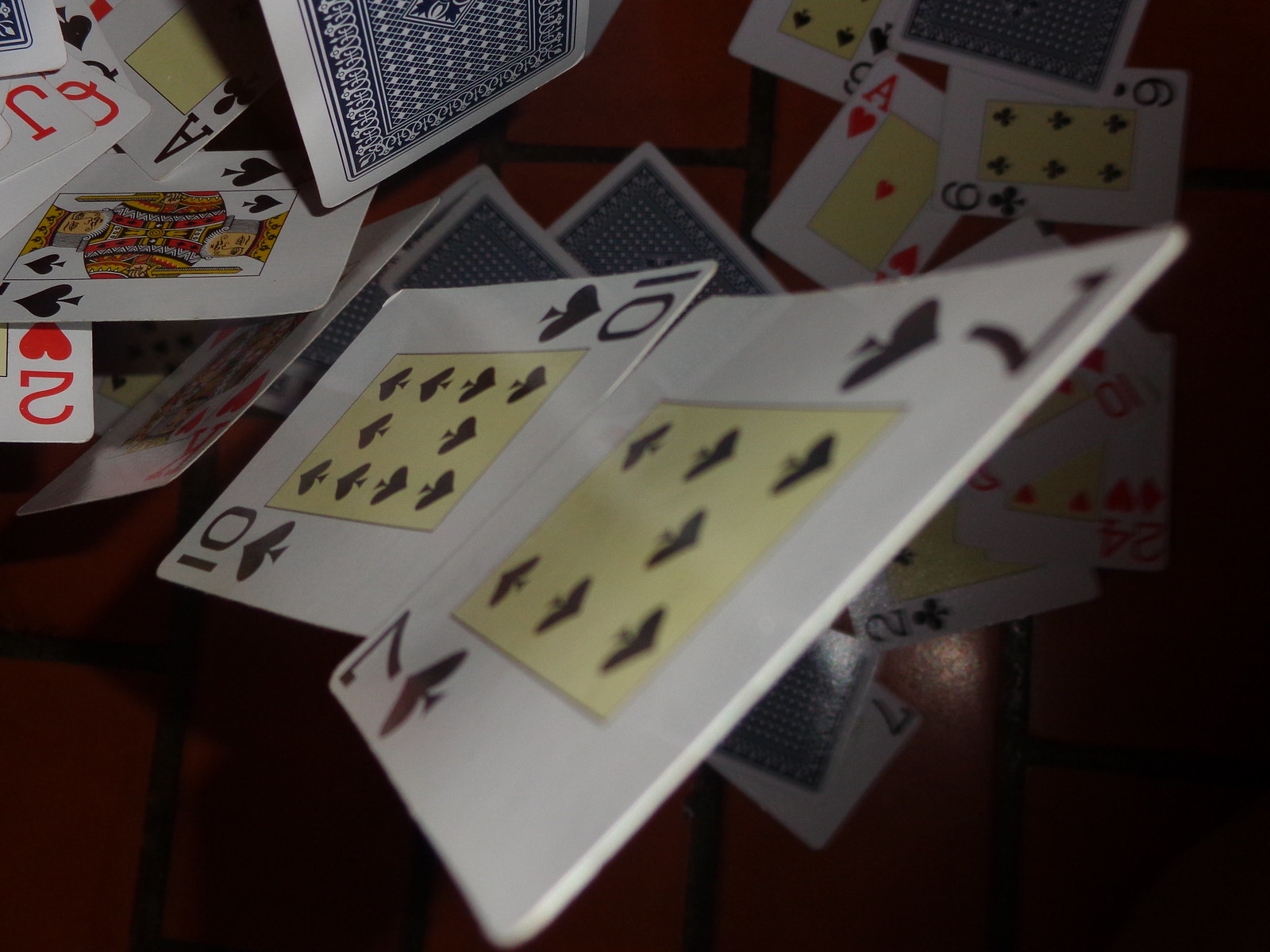This close-up photograph captures a variety of playing cards laid out on a brick surface, creating a visually intriguing scene. In the foreground, a thick, almost out-of-focus Seven of Spades takes up a significant portion of the frame, featuring a distinctive yellow rectangle pattern with spade symbols matching the card's number. Two cards, the Ten of Spades and another, are stacked vertically, appearing larger than typical playing cards. Arranged neatly on the brick surface are an Ace of Hearts, a Six of Clubs, a Six of Spades, a Two of Hearts, a Jack of Spades, an Ace of Clubs, a Red Jack, and a Red Queen. Notably, the Red Jack and Red Queen are only partially visible, showing just their corners and facing the camera. This detailed ensemble of cards set against the textured backdrop offers an interesting blend of colors, shapes, and patterns, inviting viewers to ponder the story behind the arrangement.